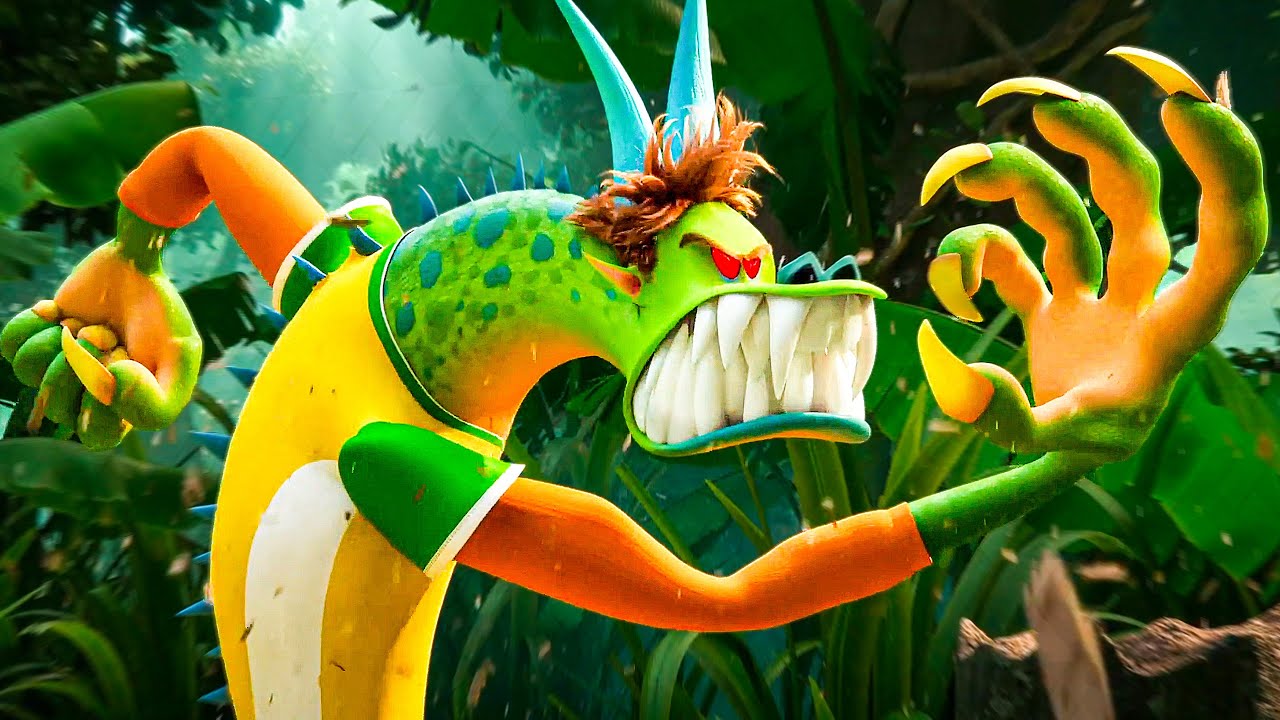This colorful and vibrant image features a detailed and menacing cartoon creature that combines characteristics of various mythical beings. The primary colors are a striking mix of greens, blues, oranges, and yellows. This humanoid monster, with dragon-like features, has green skin and an elongated, banana-shaped body clothed in a yellow shirt with green and orange sleeves, accented with a white stripe. Its grotesque face displays bright red eyes, an array of large, menacing white teeth, and a blue nose. The top of its head is adorned with blue horns and orange hair, while blue spikes trail down its back. The creature's hands are disturbingly large, featuring abnormally long, weapon-like fingernails. Posed in a combative stance with one arm behind its back and the other extended forward, it appears to be motioning to grasp something. The backdrop is an enigmatic green and black setting, suggesting a forest or underwater locale, enhancing the sense of peril and mystique surrounding this formidable monster.